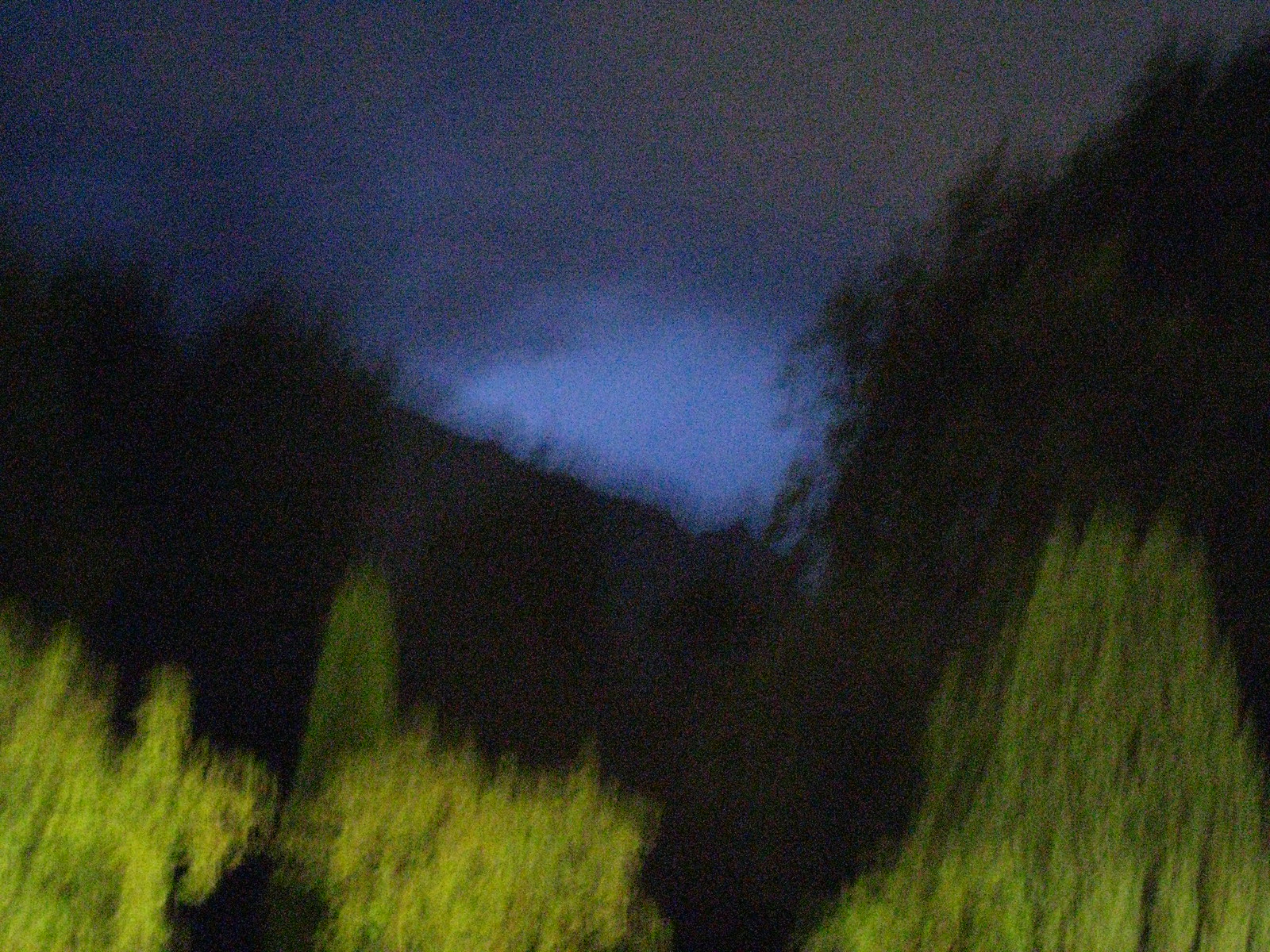This photograph captures a nighttime outdoor scene that appears to be taken at dusk in a forest or a heavily wooded area. The sky is predominantly dark, transitioning from black at the edges to a lighter blue and purple as it descends towards the center, forming an arched, slightly lit half-circle in the middle. Blurry silhouettes of trees and their leaves form a striking V shape, darkened to the point of appearing completely black due to the lack of light. In the foreground, noticeable yet very blurry, are bright green and yellowish bushes or possibly pine trees, with their tops faintly illuminated. These foreground plants, including some cypress-like greenery, add a touch of light green amidst the dark, shadowy backdrop, making the scene appear as though it's on the cusp of twilight.